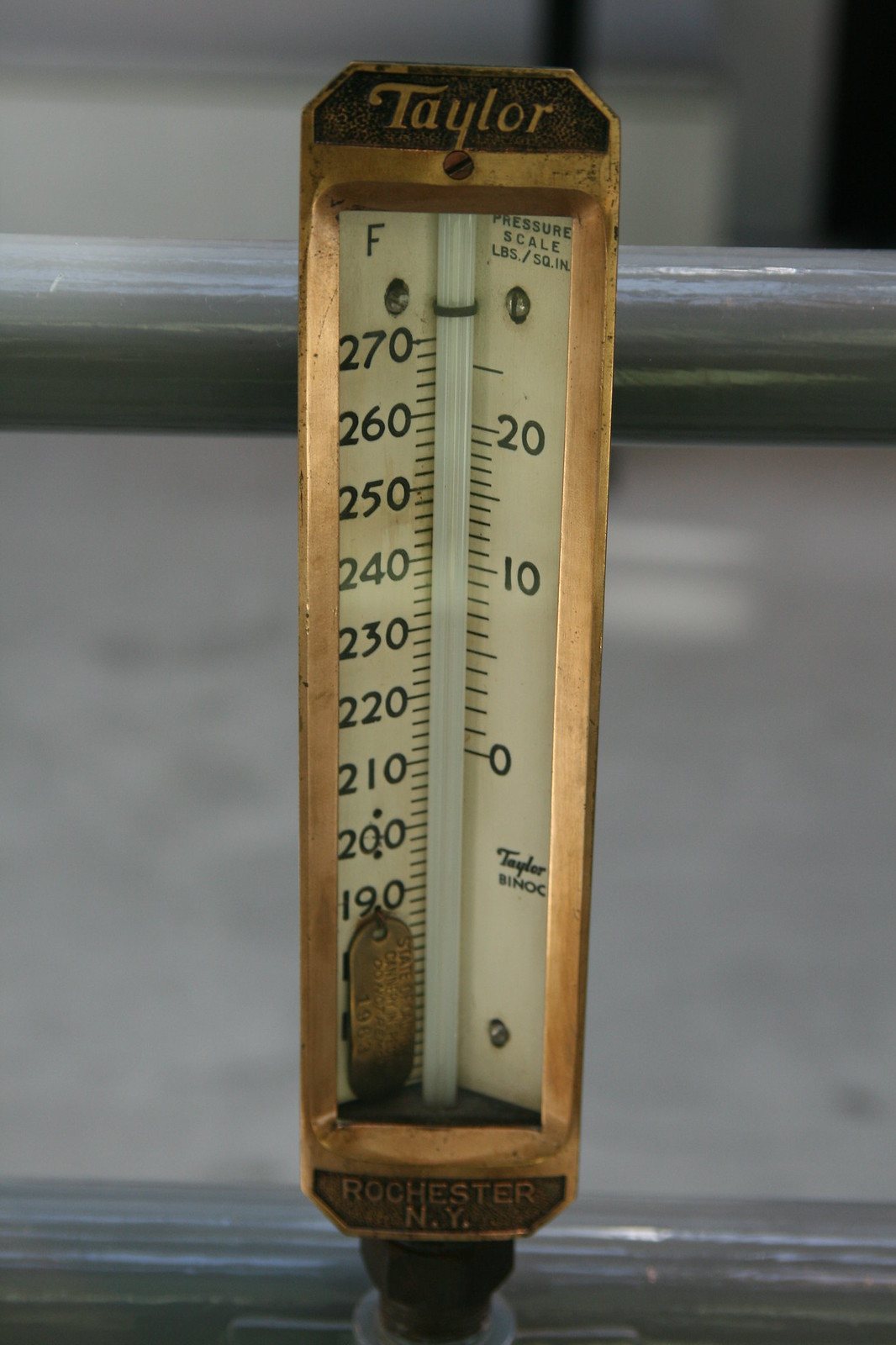This photograph showcases a vintage brass thermometer, possibly of industrial use, mounted on a vertical pipe with a hexagonal bolt at the base. The device appears to be quite old and carries the brand name "Taylor" inscribed at the top, with "Rochester, New York" noted at the bottom, indicating its place of manufacture. The image reveals a gray horizontal line at the bottom and an out-of-focus white surface in the background, suggesting the photograph was taken in an indoor setting, possibly within a machine room or a similar environment.

The left-hand side of the thermometer features a temperature gauge marked with "F" for Fahrenheit, ranging from 190°F to 270°F. Partially obscured by a brass component at its lower section, the scale is clearly visible higher up. On the right-hand side, there is a smaller pressure scale measuring in pounds per square inch (psi), with increments marked from 0 to 30 psi, and smaller gradations in between. Together, these elements suggest the thermometer was designed to monitor temperature and pressure, likely in an industrial setting.